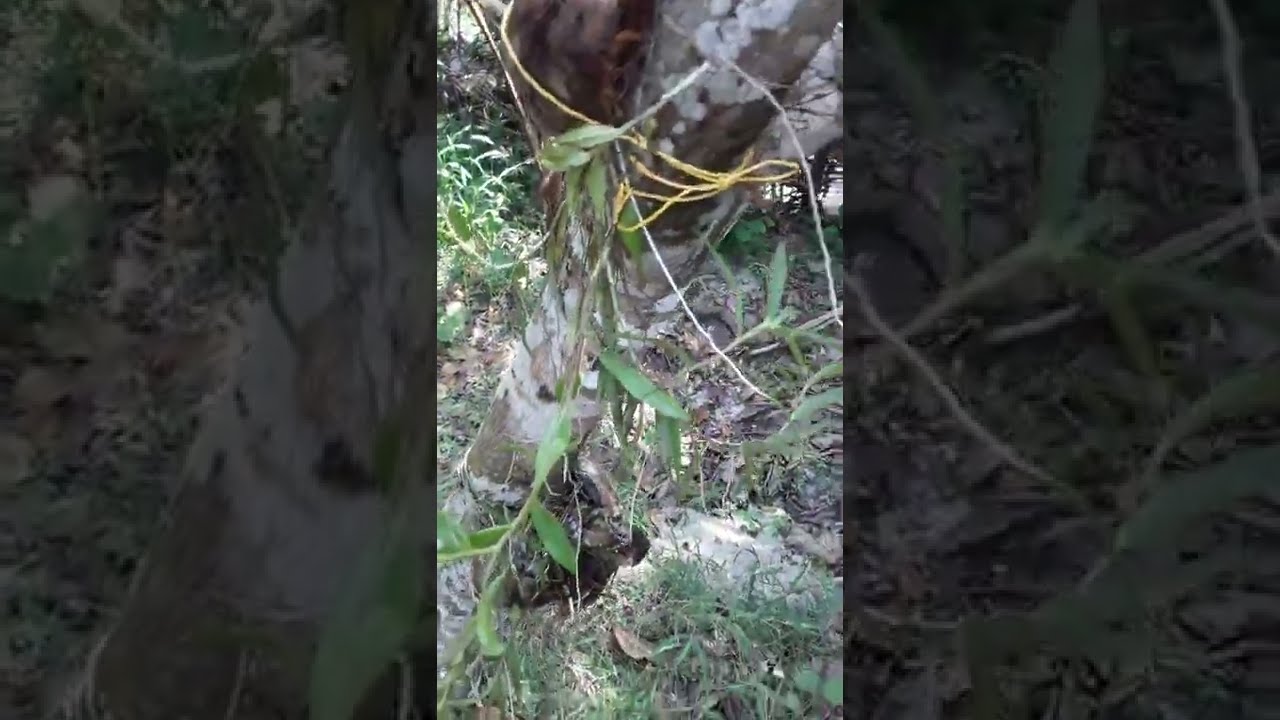In the foreground, the image depicts a tree with a blend of white and brown hues, adorned with trailing vines and a yellow twine tied in a bow near the top. The ground is speckled with grass and dead leaves, with small twigs scattered around, possibly intertwined with the vines. The setting, illuminated by daylight, reveals the intricate textures on the tree trunk, which is cloaked in varying shades of dark gray and hints of rust. This image is superimposed over a larger, zoomed-in version of itself, which serves as a shadowy backdrop, creating a camouflage effect with its muted browns and greens. A mysterious hole at the tree's base is partly obscured by long vines, leaving it unclear whether it shelters an animal. The overall composition is vivid in the center but fades into dark shadows at the edges, encapsulating the natural scene in an almost surreal ambiance.